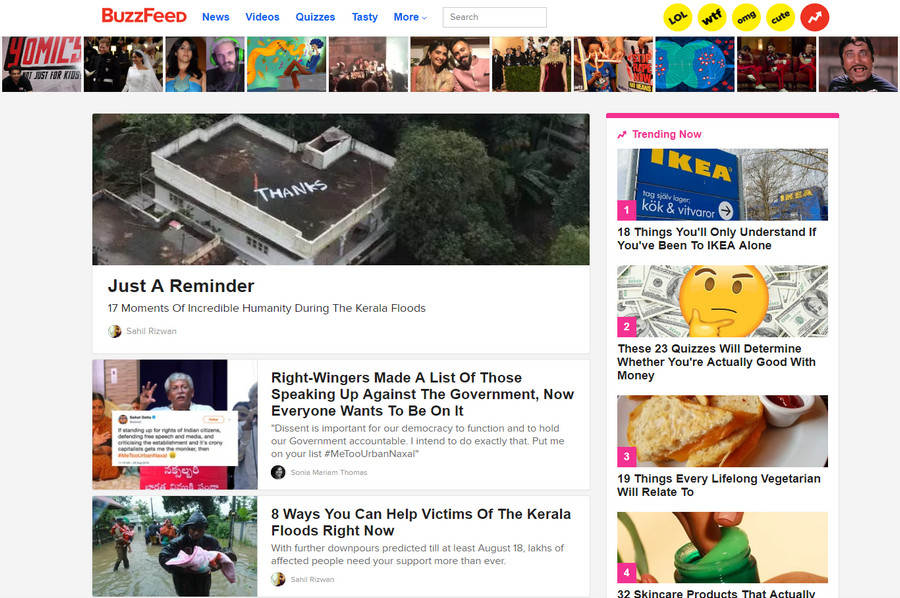This screenshot captures the BuzzFeed homepage with a clear and structured layout. At the top-left corner, the BuzzFeed logo is prominently displayed in red font. Adjacent to the logo, a blue navigation menu offers categories: News, Videos, Quizzes, Tasty, and More, followed by an empty search box. 

Next to the search bar, there are five interactive circles: four yellow ones labeled LOL, WTF, OMG, and CUTE, and one red circle featuring a white arrow. Below this navigation, a horizontal row showcases various images of people, likely including actors and celebrities.

The main story, titled "Just a Reminder: 17 Moments of Incredible Humanity During the KERALA Floods," features a photo of a building with "thanks" painted on its roof. This is succeeded by additional images: one depicting a man and another of an individual navigating floodwaters while holding a child.

To the right, a section lists the top four trending stories, inviting further exploration.